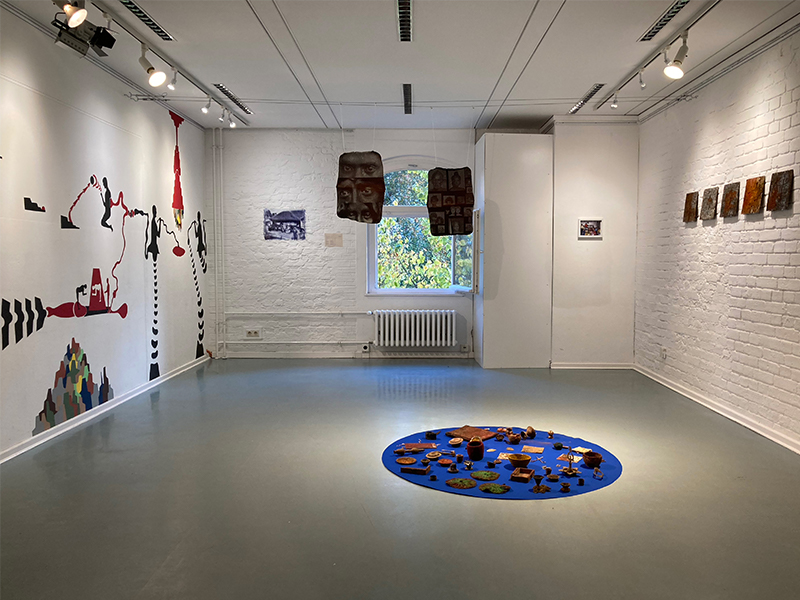The room is an eclectic blend of traditional and contemporary design elements. On the left side, the wall is painted sheetrock, adorned with a variety of artistic scenes in hues of blue and red. The far wall directly ahead features a white-painted brick exterior, punctuated by a centrally placed window. Below the window is a traditional radiator, and to its side stands a cabinet. In the corner, there is a built-in structure, possibly part of the heating system.

The right wall displays a mix of rough and regular brickwork, all uniformly painted white. Lined along this wall are five paintings of the same size but in varied colors: dark brown, gray, another brown, a reddish hue, and yet another shade of brown. These paintings are meticulously hung at equal height.

The floor is covered in gray linoleum, in the center of which is a conspicuous blue dot, surrounded by what appears to be miniature army men, arranged in a strategic setup. Overhead, track lighting illuminates the room, with interesting suspended rock-like sculptures hanging from the ceiling. The overall decor blends artistic creativity with functional elements, creating a visually stimulating environment.